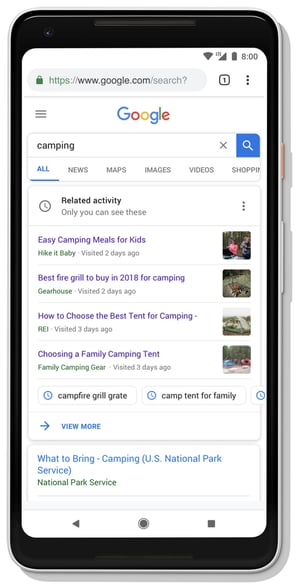The image shows a smartphone screen displaying the Google search engine homepage. In the search bar at the top, the query "camping" is typed. Beneath the search bar, a message reads, “Related activity: Only you can see these.” Below this message, the first search result is titled “Easy camping meals for kids.” Following this, several other blue links appear sequentially, each pertaining to camping-related topics. The subsequent links are listed as: “Best fire grill to buy in 2018 for camping,” “How to choose the best tent for camping,” “Choosing a family camping tent,” and the last link at the bottom of the screen reads, “What to bring camping – U.S. National Park Service.”